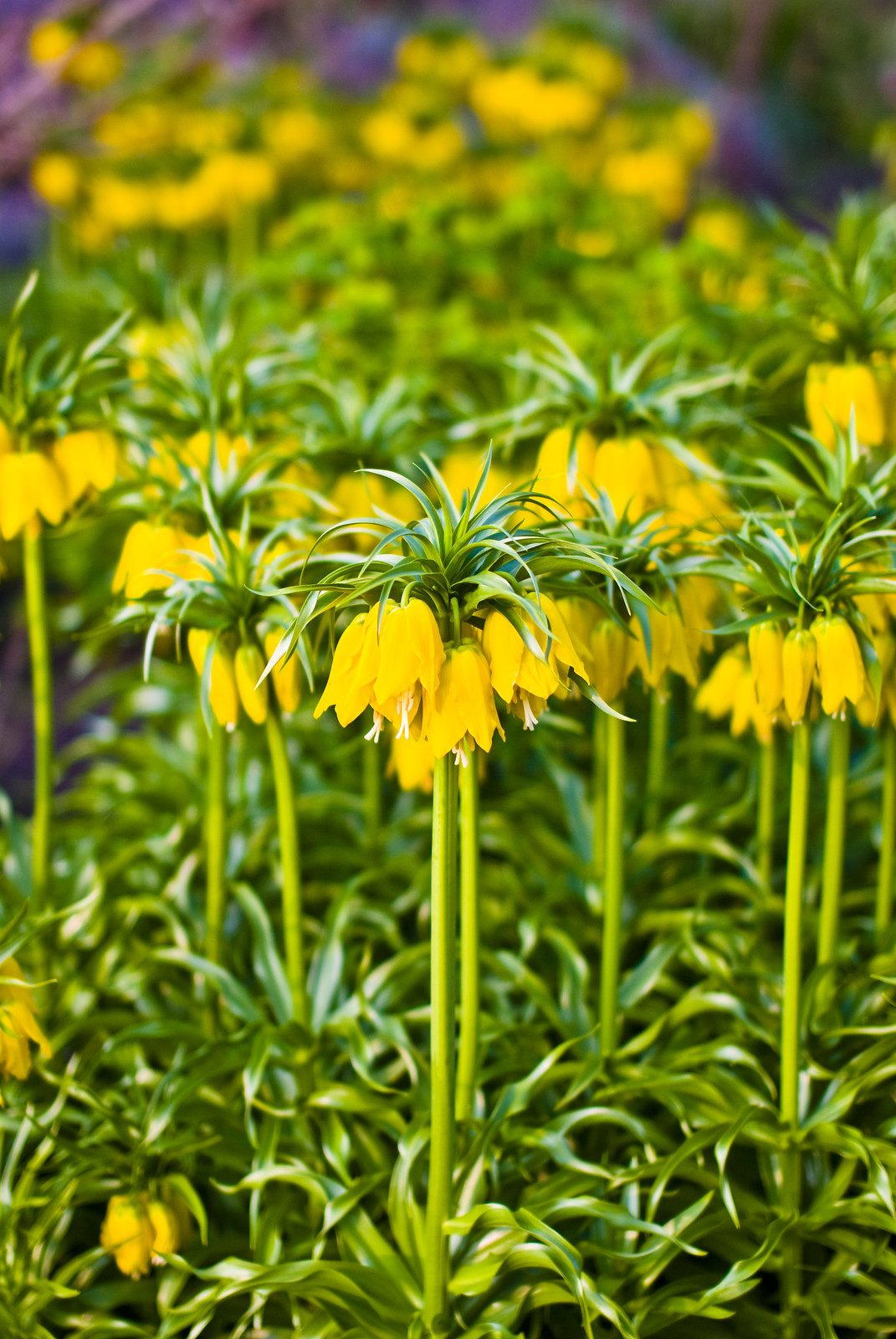In this detailed image, the foreground is sharply in focus, showcasing a sea of yellowbell flowers, identifiable by their clusters of drooping yellow petals. Each flower emerges on a long green stem rising from a lush bed of leaves that carpet the ground. The flowers are not fully blossomed, with yellow petals hanging down and green sprouts extending above the clusters. Some thin, small palm-like leaves droop over the flowers, with white stringy filaments visible in the center of the blooms. The background is out of focus, fading into a blur of yellow clusters, giving the scene an ethereal continuity. The entire composition portrays a dense, vibrant field of yellowbells, despite some uncertainty about the exact species, capturing their characteristic appearance beautifully.